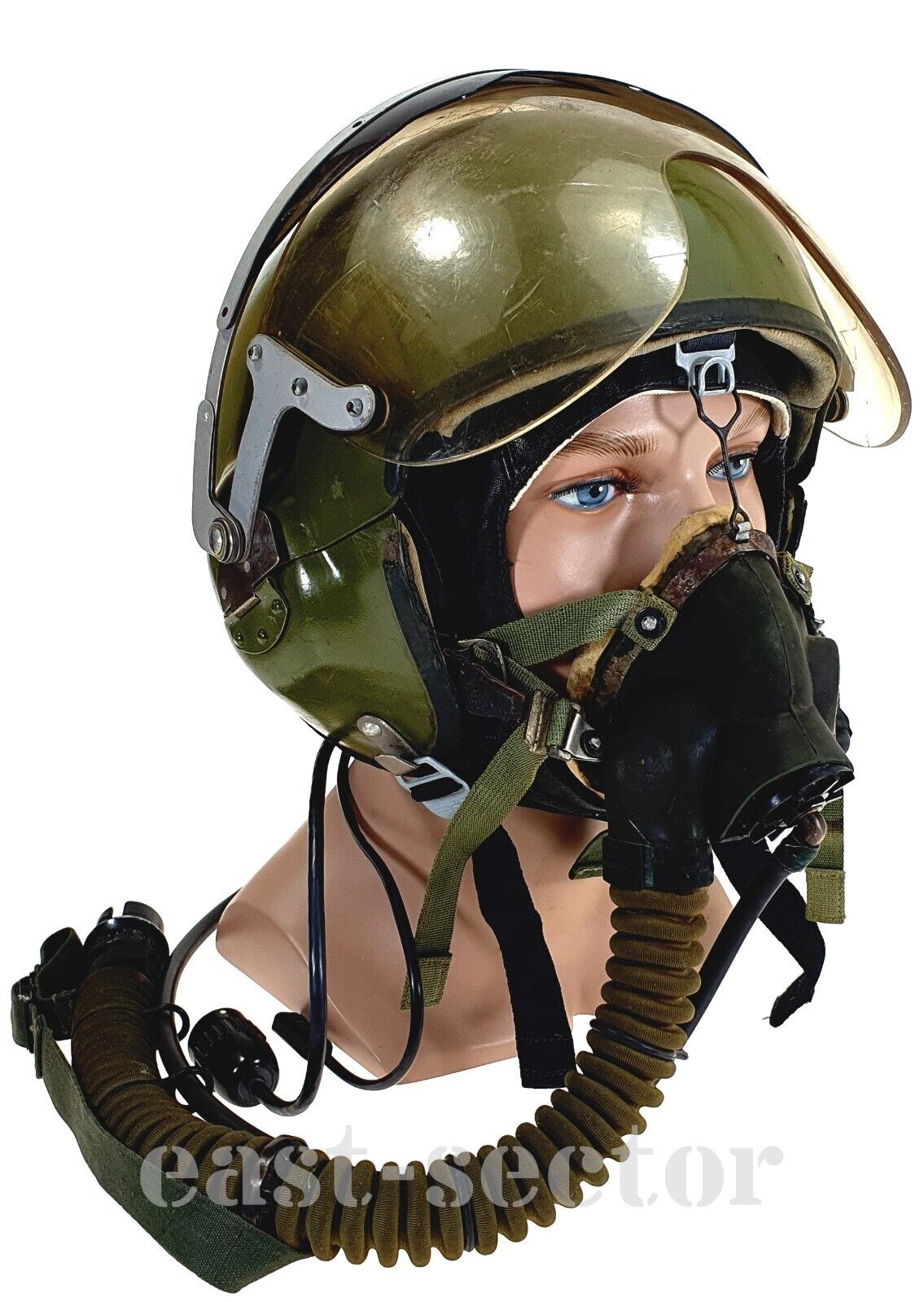This photograph features a detailed depiction of a mannequin adorned in a fighter jet pilot's headgear, complete with an olive-green helmet and a respirator. The helmet, of a traditional military olive-green hue, covers the ears, top of the head, and back of the neck. It features a thick, plastic visor flipped up to reveal the mannequin's painted blue eyes. Attached to the helmet are a couple of black wires and various metal buckles, as well as dark green straps that connect the respirator to the helmet.

The respirator, covering the mannequin's mouth and nose, is primarily black with a whitish-yellowish soft lining to ensure comfort. A large, dark brown flexible air hose extends from the respirator, wrapping around the mannequin and suggesting connection to an oxygen system. The mannequin itself is white, with a focus primarily on the head and neck areas, making the equipment the central feature of the image. The scene is set against a plain white background with a watermark at the bottom that reads "East Sector," hinting at possibly a military instruction guide or stock photo.